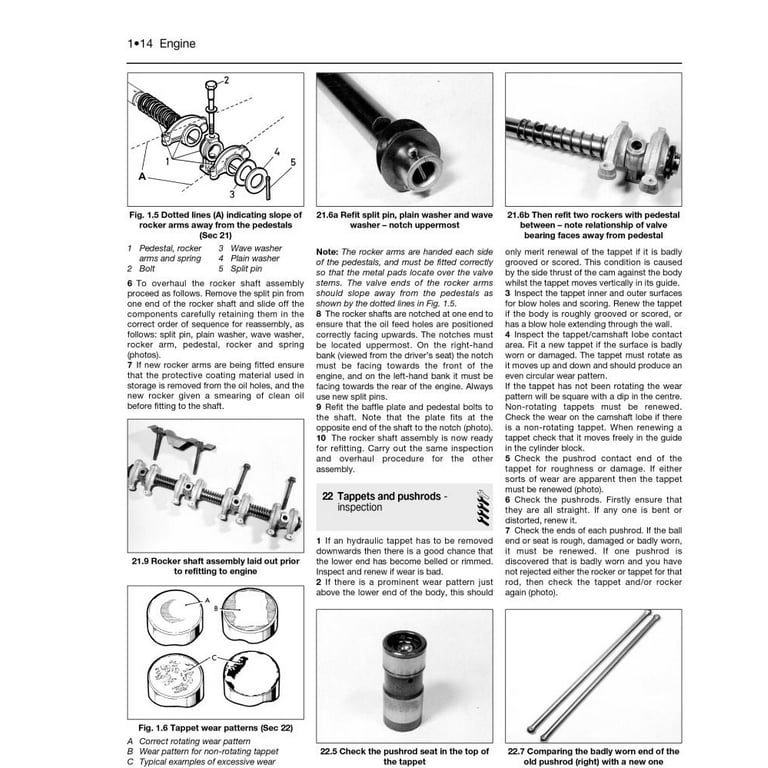This image captures a detailed page from an instruction manual specifically for a vehicle's engine. The top of the page is labeled "1.14 Engine," and it comprises three columns filled with text and images. The page includes diagrams and photographs labeling various engine components with intricate details. Notable figures include "1.5," depicting a part of the engine with a dotted line marking the top of the locomotive away from the pedestal, and "2.16A," which references a split pin plain washer with a wave washer notch uppermost. "2.16B" features two locomotives with a pedestal between them. Key parts such as rocker arms, split pins, bolts, tappets, and pushrods are explicitly described, highlighting their roles and interplay within the engine assembly. Detailed instructions guide the reader on checking the pushrod seat in the tappet's top and examining tappet wear patterns. The comprehensive documentation ensures each part is thoroughly identified and its function clearly explained, contributing to an in-depth understanding of engine mechanics.